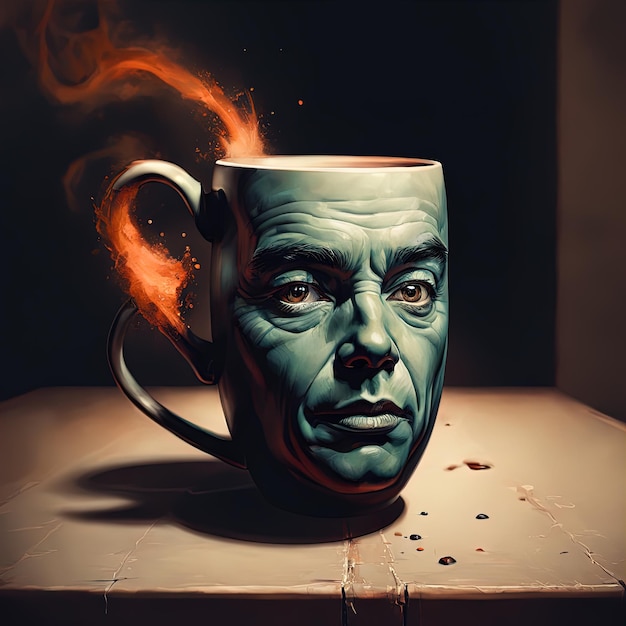This digital creation depicts a prominently featured, tall, ceramic coffee mug set against a black backdrop, with a subtle gray wall on the right side. The mug, placed on a rustic, possibly wooden table marred by cracks and imperfections, stands out due to its unusual design. The mug showcases a photorealistic face of an old man with deep wrinkles and tired, brown eyes on its side. It's unclear whether the face is merely printed on or if the mug is shaped into the facial contours. Intriguingly, the mug possesses two vertically aligned handles on its left side. Flames emerge from both the top of the mug and one of its handles, casting an eerie glow. The grayish-blue hue of the mug contrasts with the vivid orange and red flames licking its surface. Adding to the surreal scene, a few drops of what seems to be blood are scattered on the table.